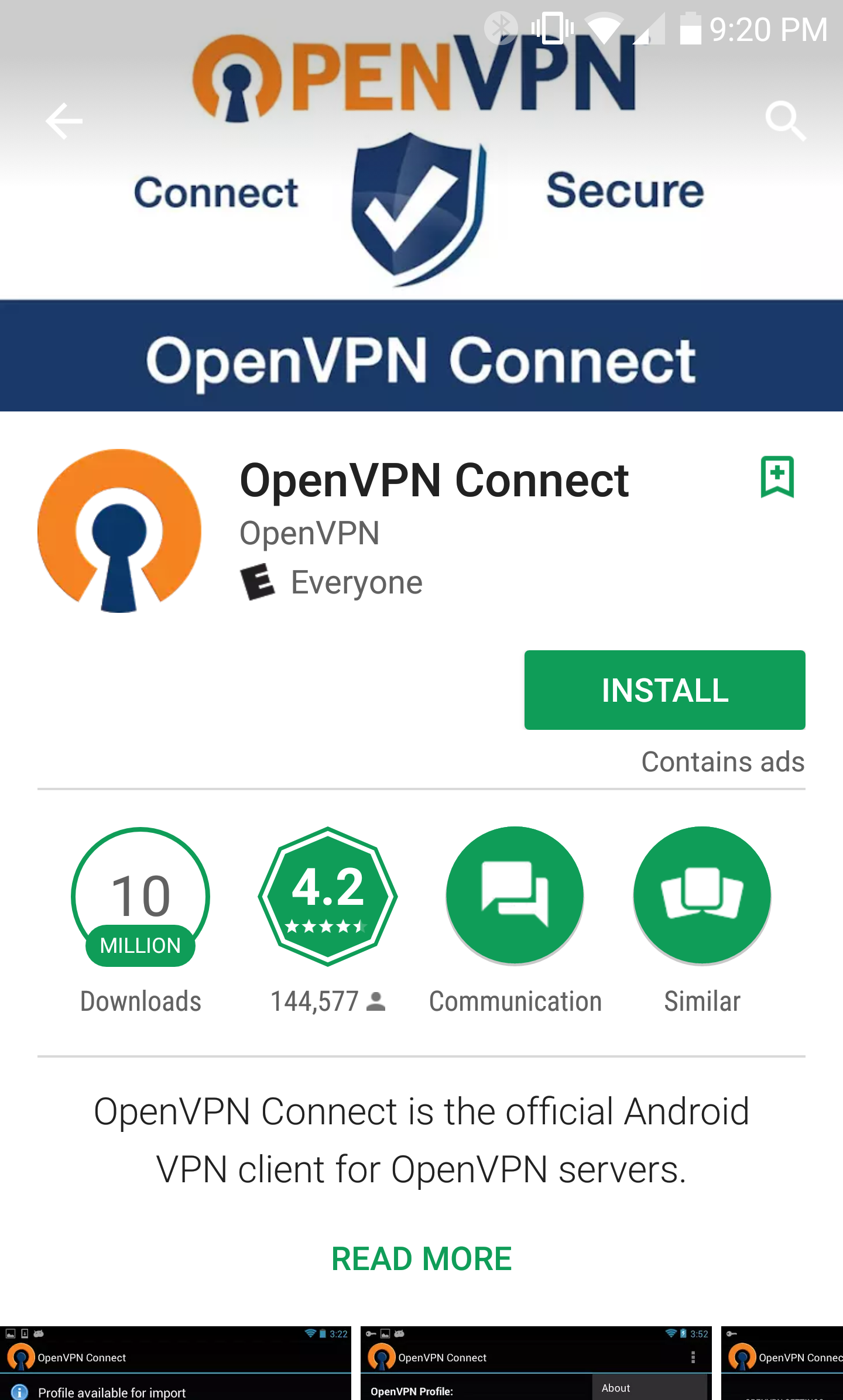This image is a cell phone screenshot displaying a website for OpenVPN. At the top center of the image, the website's logo is prominently featured. The logo consists of the letter "O" in orange with a blue keyhole at the bottom, followed by the letters "PEN" in orange. To the right, the letters "VPN" are capitalized and displayed in dark blue.

Beneath the logo, to the left, there is a left-facing white arrow, and to the right, a white magnifying glass icon. Below these icons, the word "connect" is displayed in blue on the left side. In the middle, there is a dark blue shield with a white trim and a white check mark in the center. To the right of the shield, the word "secure" is written in blue. 

Further down, there is a dark blue rectangle containing the text "OpenVPN Connect" in white letters. Below this, toward the left, the logo appears again, showing the "O" with its top portion in orange and the keyhole area in dark blue. To the right of it, "OpenVPN Connect" is written in black letters. Adjacent to this, there is a plus flag symbol.

Moving lower, on the left, the text "OpenVPN" is written in gray, and underneath this, the letter "E" is in bold black with the word "everyone" in gray to its right. On the right, there is a green button with the word "install" in white. Beneath this button, the text "contains ads" is displayed in gray.

Further down, there is a circular icon with a green border and a white center containing the number "10" in gray. Below this circle, the word "million" is written in white. To the right, there is a green hexagon with a white "4.2" inside it, and beneath it, "4.2 stars" in white. Further right, there is a circle with two white message boxes, followed by another circle containing three white squares.

At the bottom, the text "OpenVPN Connect is the official Android VPN client for OpenVPN servers" is written in gray. Below this, a green "read more" button is prominently displayed in the middle. On the bottom left, middle, and right of the screen, there are black bars with writing that is too small to be legible.